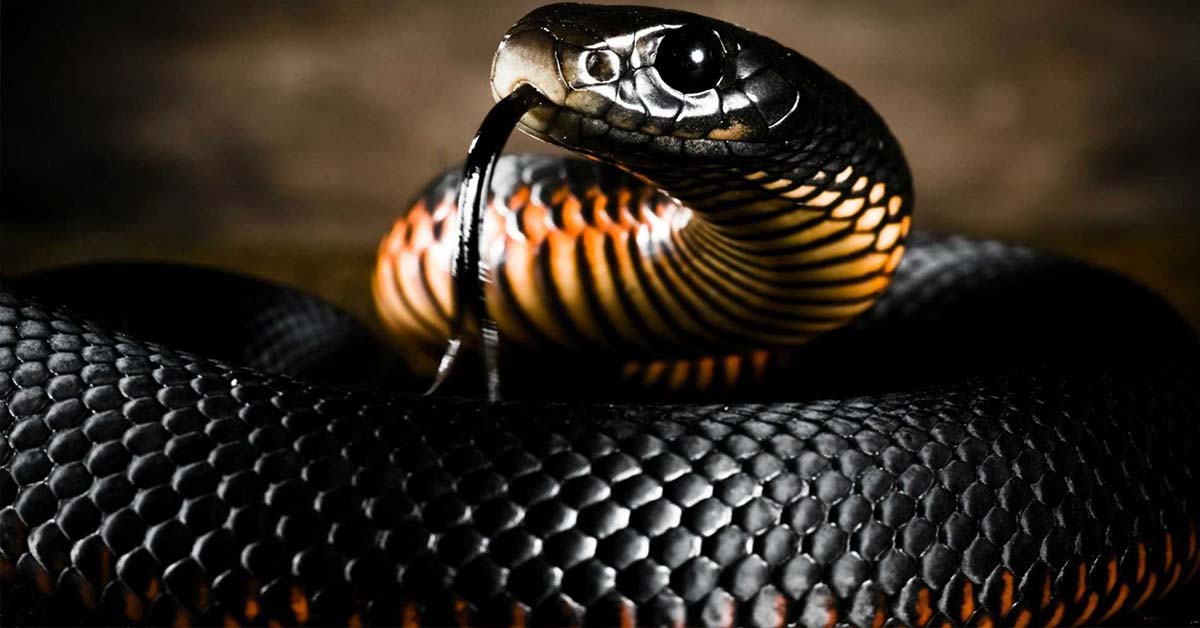This professionally shot, studio photograph captures a striking close-up of a black python, dramatically curled around itself. The snake's head, positioned at the top center of the image, features a large, dark eye with a slight white reflection from the studio lights, enhancing its shiny appearance. The python's tongue, deeply black and forked at the end, protrudes from its closed mouth. The scales across its body are prominently black, while underneath, the snake displays alternating horizontal stripes of light orange-yellow and black, giving it a unique and textured look reminiscent of an armadillo's armor. The background is shaded brown, providing a stark contrast to the python’s dark scales and further emphasizing the intricate details of the snake's reptilian skin. The photo is landscape-oriented, approximately twice as wide as it is tall, and offers a detailed view of the python's natural beauty, devoid of any text.